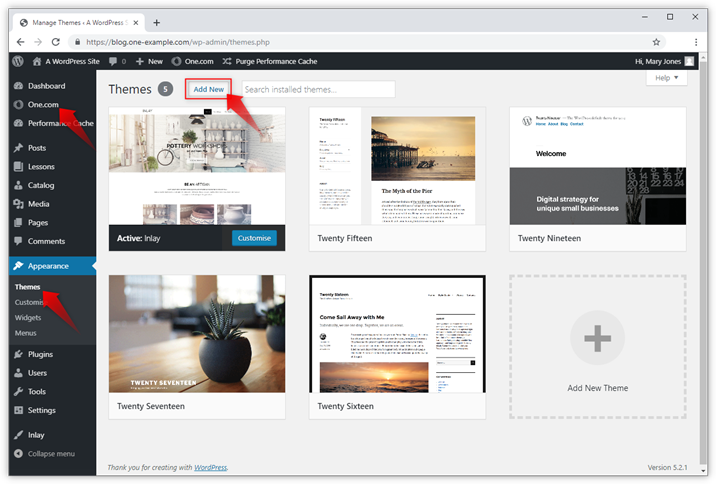The image is a screenshot of a WordPress website's "Manage Themes" page. In the top left-hand corner, you can see one browser tab open, titled "Manage Themes for WordPress." The interface showcases a section dedicated to managing website themes.

On the left side of the interface, there is a vertical black sidebar featuring navigation options. Notably, three red arrows highlight important areas on the screen:
1. The first arrow points to a "Themes" button, likely used to access the theme management section.
2. The second arrow highlights a link labeled "One.com," indicating a website service or provider.
3. The third arrow points to an "Add New" button, which is white in color and allows users to add a new theme.

The main area of the page displays five distinct theme options available for selection, each with a name and thumbnail. The themes are titled "Twenty Fifteen," "Twenty Nineteen," "Twenty Seventeen," "Twenty Sixteen," and one more not specified in the description. The overall background of the interface is predominantly white with contrasting elements for clarity and organization.